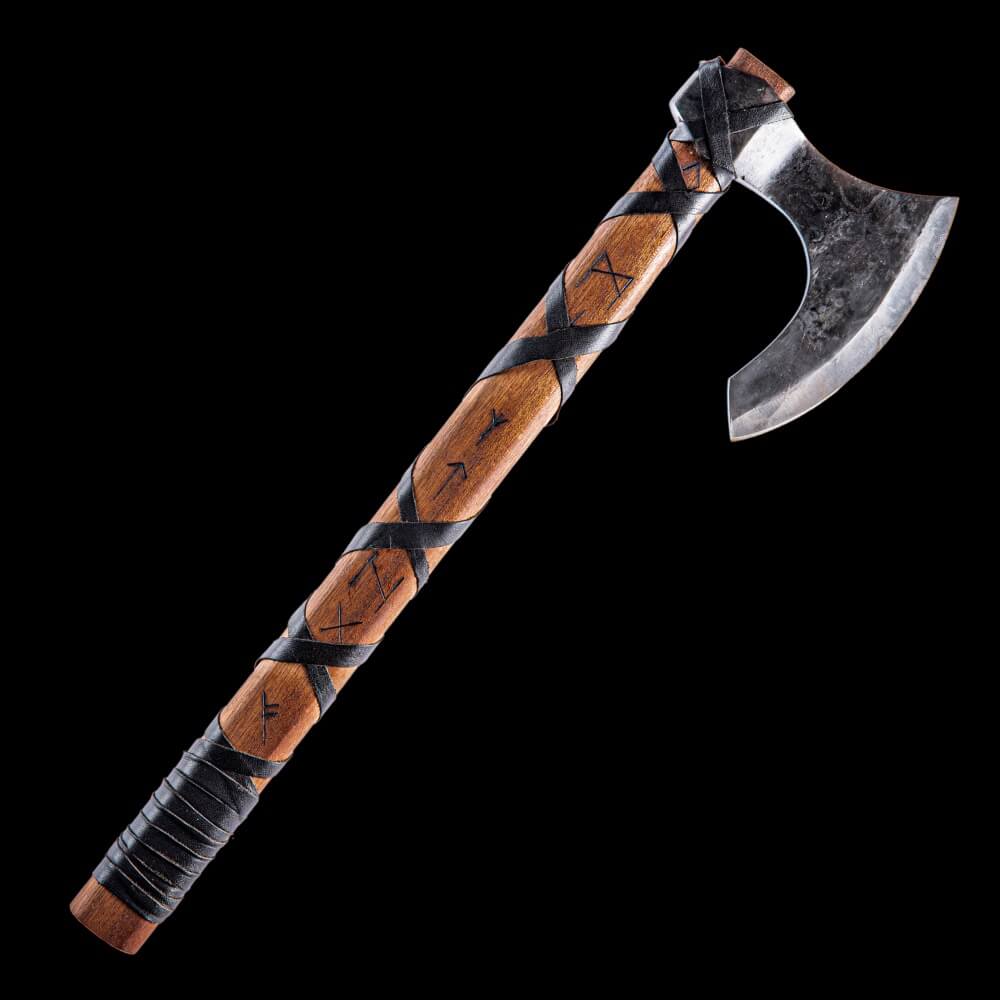In this captivating image set against a solid black background, a striking hatchet takes center stage. The hatchet features a robust wooden handle, intricately adorned with a black tape design. Along the length of the handle, precisely crafted black tape is wrapped, interspersed with four prominent X-shaped markings, adding a rugged yet artistic touch. The blade, reminiscent of a tomahawk yet more akin to a modern hatchet, showcases a unique U-shaped or semi-U-shaped carving, blending functionality with distinctive styling. The overall composition presents a compelling blend of traditional craftsmanship and contemporary design.